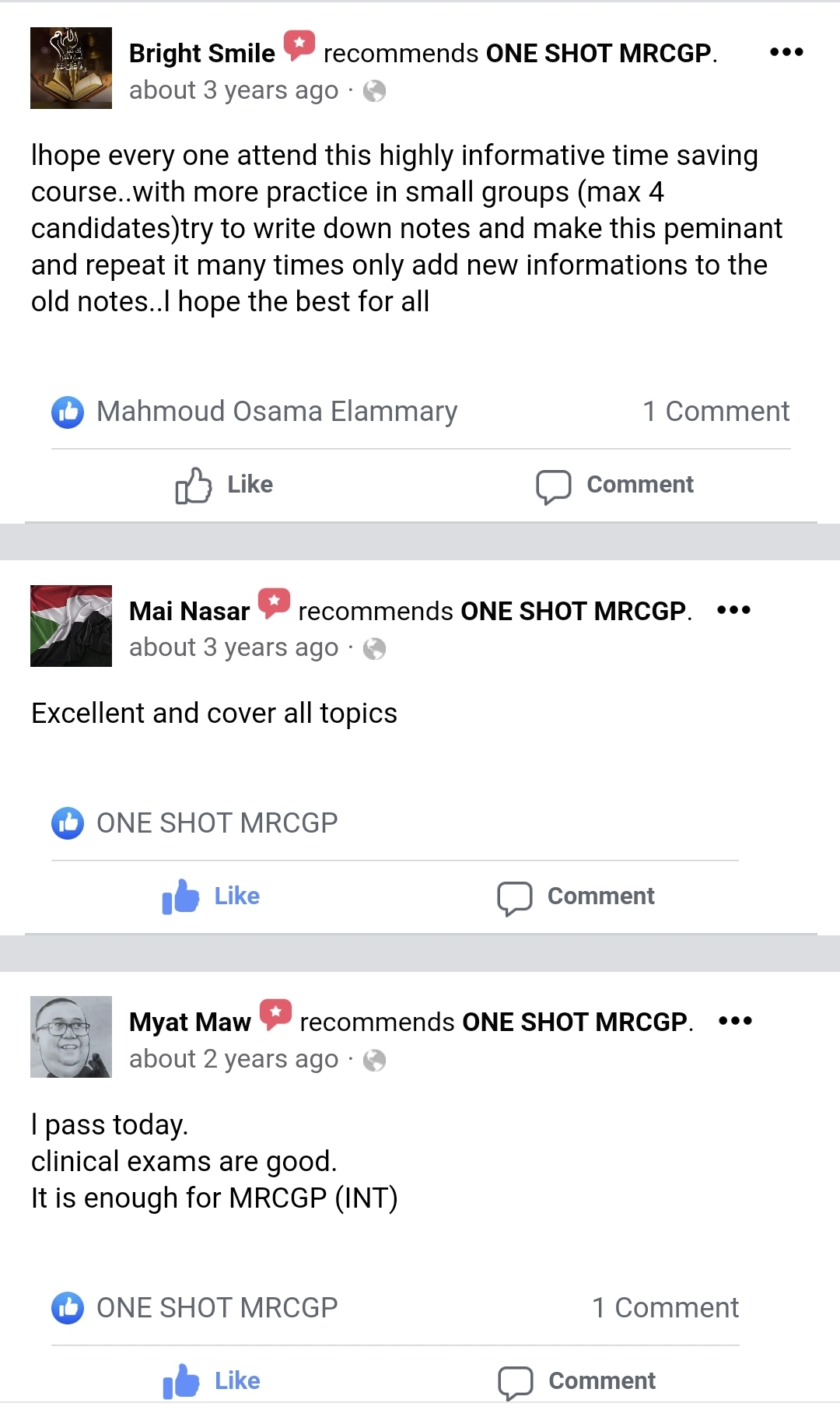Here's a cleaned-up and detailed caption for the image described:

---

The image showcases a series of posts from what appears to be a discussion forum or a review section on a website. The posts primarily discuss a course called "One Shot MRC GP" and include recommendations and experiences from different users over the years. 

**Top Post:**
A bright, smiley icon accompanies a recommendation for the "One Shot MRC GP" course from about three years ago. The user Muhammad Osman Almar describes the course as highly informative and time-saving, emphasizing the benefits of practicing in small groups with a maximum of four candidates. He advises taking detailed notes and updating them with new information regularly for better retention. His well-wishes conclude the post, which has garnered one comment.

**Middle Post:**
Another user, possibly named MAI NASCAR, also recommends the "One Shot MRC GP" course from three years ago. Their brief but positive comment highlights that the course is excellent and comprehensive, covering all required topics. This post is marked with a blue light, indicating its importance or positivity.

**Bottom Post:**
The final post shows Matt M and My a T Ma M a W sharing their success story from two years ago. They mention passing their clinical exams and question if it is sufficient for the MRC GP (Member of the Royal College of General Practitioners) certification. Like the middle post, this one also has a blue light and has received one unseen comment.

The color scheme of the platform includes black, white, gray, red, orange, green, and blue, with the blue lights possibly signifying positive feedback or notable comments.

---